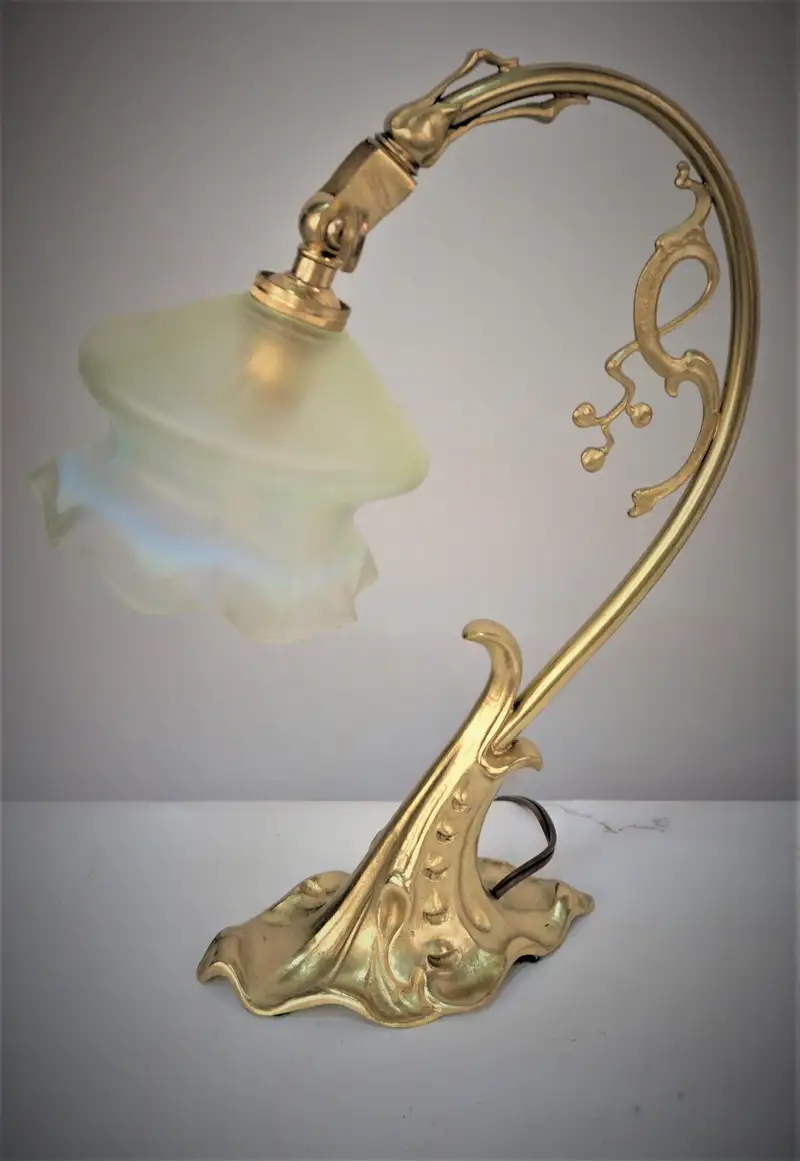This is an up-close image of an ornate lamp set against a pure white wall and resting on a white table. The lamp boasts a detailed, elaborate gold base, which resembles an upside-down flower with a wavy, draping design. From this base extends a polished gold pole that sweeps upward and to the right before curving back in a reverse C shape. Within this curve, a smaller S-shaped gold piece adds to the intricate design. The lamp culminates in a frosted glass light cover, which takes the form of a mushroom top, featuring fluted edges that give it an elegant, flower-like appearance. A barely visible black cord trails down from the lamp, adding a subtle modern touch to its overall vintage aesthetic. The lamp's design, with its flowing curves and decorative elements, exudes an old-world charm, making it a standout feature in the room.